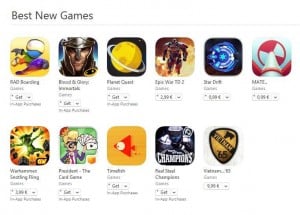The screenshot features a selection of the best new games, with a crisp white background. At the top of the image, there are three distinct game icons prominently displayed, though the specific titles are unreadable. Below these, five additional game icons are aligned, also without discernible text. To the left side of the image, the phrase "Best New Games" is indented, adding an organized touch to the presentation.